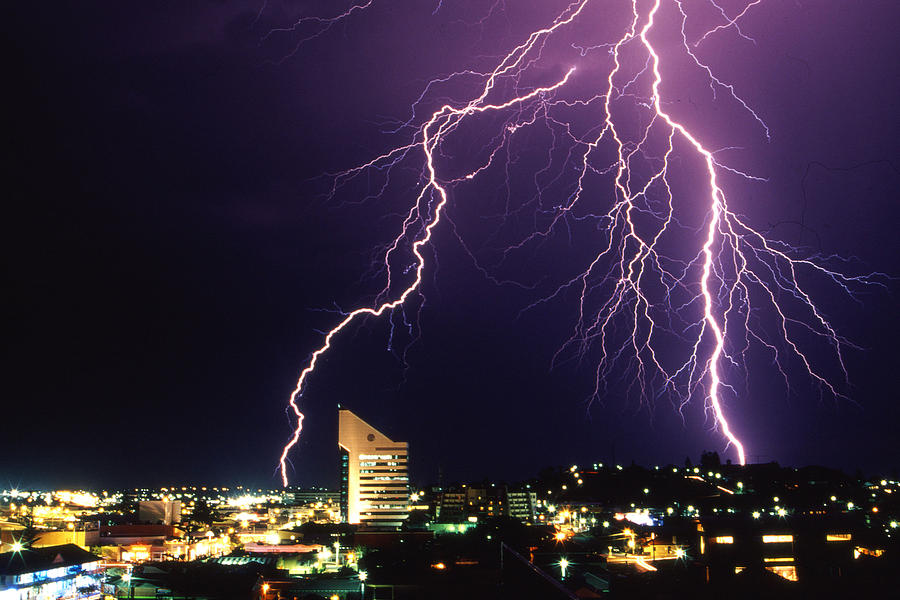This nighttime photograph captures a dramatic lightning strike illuminating a large cityscape. The city occupies about a sixth of the frame along the bottom edge, its skyline dominated by numerous lit-up buildings, primarily low-rise structures with one notable multi-story building at the center featuring a distinctive sloping roof. Above the city, the sky transitions from very dark navy blue to lighter neon blue and purple hues surrounding the lightning strike. The lightning itself is thick and elaborate, with several prominent white branches and a complex network of smaller vein-like tendrils radiating outwards. The scene suggests an impending fierce storm, with the striking contrast between the brightly lit city and the electrified, stormy sky above.